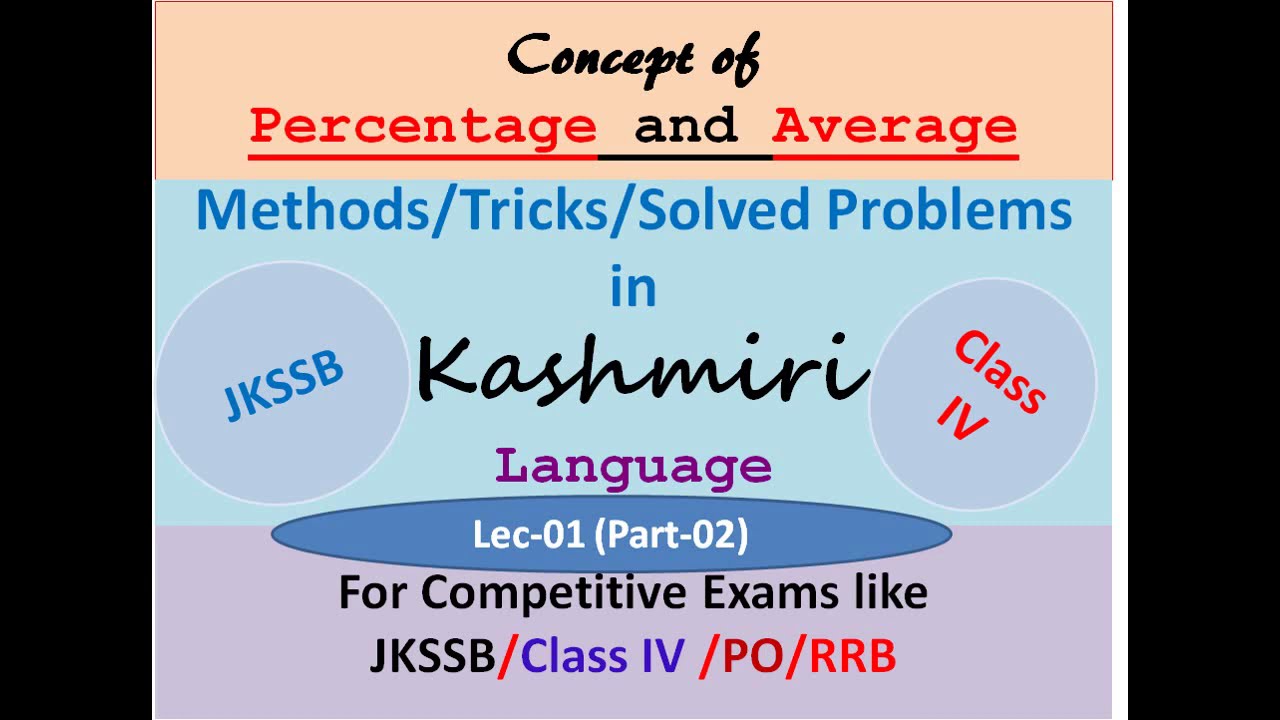The image features a horizontally aligned rectangular layout with thick vertical black borders on both sides. At the top of the image, set against a beige background, is the title "Concept of Percentage and Average," with "Concept of" printed in black and "Percentage and Average" in red, emphasized by black underlining. Below this, the middle section has a blue background and contains the text "Methods / Tricks / Solve Problems" followed by "in Kashmiri," with "Kashmiri" in black and "Language" in purple. In the center, the word "CASMIRI" stands out in black text. Flanking this central word, on the left side is a gray circle labeled "JKSSB" in blue, and on the right side is a similarly shaped circle that says "Class 4" in red, signifying the enrollment number. At the bottom, there is a light purple section reading "For competitive exams like JKSSB / Class 4 / PO / RRB" in black text.